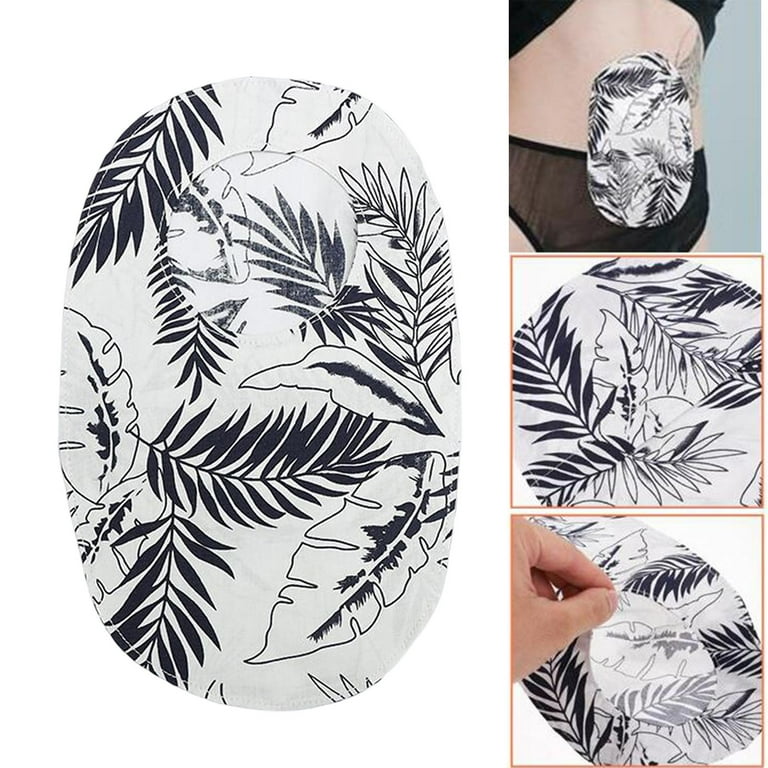This image features a detailed black and white oval-shaped design with various types of palm and fern leaves, set against a white background. On the left side, the main design prominently displays the intricate leaf patterns. To the right, a vertical column showcases three progressive images with orange-outlined borders. The top image illustrates the oval fabric applied to a person's torso, likely a woman in underwear, covering her stomach and partially over the underwear, suggesting the use of this fabric as a tattoo stencil. The middle image provides a close-up view of the fabric's detailed leaf patterns. The bottom image captures a hand peeling the fabric, indicating the removal process of the stencil after applying the ink. This series of photos demonstrates the application and function of the stencil template for tattooing.